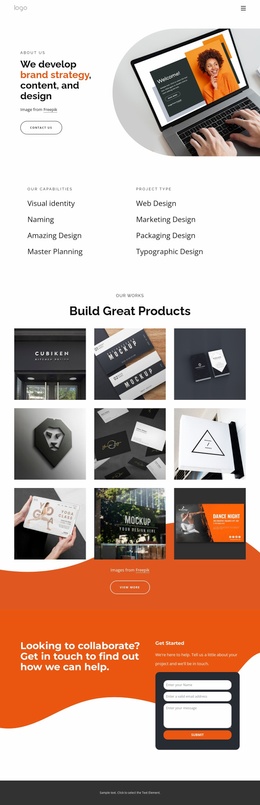This image is a full-page screenshot of a brand consulting company's website, displayed in a mobile landscape format, which allows the entire page to be viewed without the need to scroll. The background is predominantly white, providing a clean and professional look.

At the top left corner, there's a brief description succinctly stating, "We develop brand strategy content and design," with "Brand strategy" highlighted in orange to emphasize its importance. 

On the top right, there is a small thumbnail image showing a person typing on a laptop, which displays a company webpage, suggesting a focus on digital engagement.

Below this section, the page is divided into two columns featuring category names. The left column and the right column each contain four categories, all written in dark gray, maintaining a uniform and minimalist aesthetic.

Centrally positioned on the page is a bold headline that reads, "Build Great Products," serving as an inspirational call to action. Directly beneath this headline, there are nine small square thumbnails, arranged in three rows of three. These thumbnails showcase a variety of company-branded products, providing a visual sample of the work and capabilities of the consulting firm.

Finally, in the bottom right corner, there is a small box with instructions on how to sign up, offering a clear and accessible call to action for visitors who wish to engage further with the company.